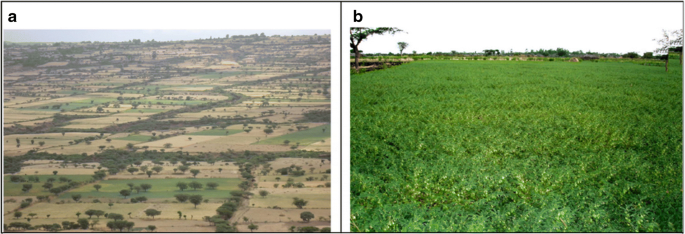The image is a composite of two color photographs positioned side-by-side in landscape orientation, each encased in a black border. In the upper left corner of the left photo, there is a black "A," and the right photo bears a black "B" in the same position. The left photograph (A) presents an aerial view captured by a drone, showcasing a diverse landscape with patches of green and dead grass outlined by rows of shrubs. There's also a light gray horizontal section near the top, possibly indicating water. The right photograph (B) offers a ground-level perspective of a grassy field, with a dense horizon of dark green trees and a few larger trees in the upper corners. This juxtaposition highlights a contrast between the aerial survey of varied terrain and the more immersive experience of standing before a lush, grassy expanse.